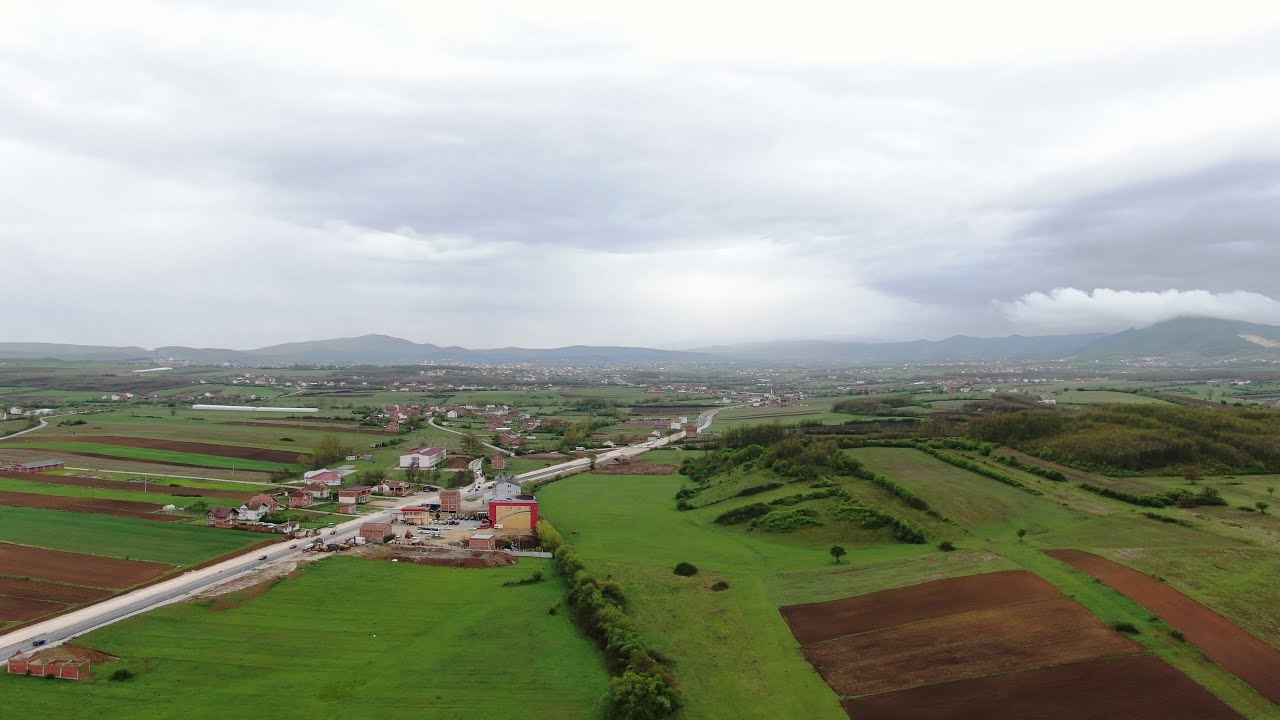This aerial photograph captures a vast, predominantly flat landscape divided equally between sky and land. The overcast sky is filled with thick, wavy clouds in shades of gray, suggesting potential distant rainfall on the horizon. The horizon itself features a not-too-tall mountain range. Below, the expansive grassland is punctuated by occasional rolling hills towards the right, adorned with short bushes and trees. The terrain also includes brown rectangular farm fields, which are interspersed with patches of greenery. A diagonal road cuts through the image, dotted with cars, and surrounded by clusters of buildings and signs of commercial activity. Further out, small white spots likely indicate houses scattered across the distance. Despite the breadth of the scene, the primary focuses are the central road, the sprawling green fields, and the contrasting brown patches of farmland.